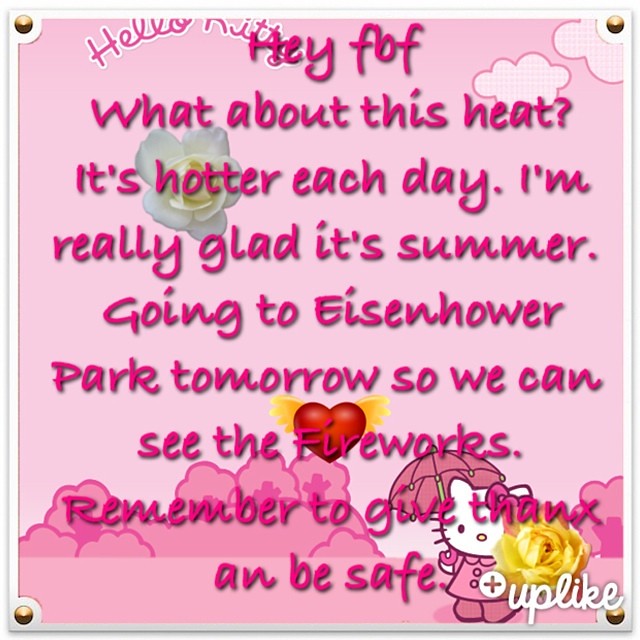This image features a detailed illustration of Hello Kitty dressed in a pink rain poncho and pink boots, holding a pink umbrella with a yellow flower adorning it. She is located in the bottom right section. The backdrop is predominantly pink, showcasing a landscape with pink ground, trees, bushes, and mountains. The sky, also in hues of pink, includes clouds and a floating red heart with yellow wings. There is pink text at the top with a shadow effect that reads: "Hey FBF, what about this heat? It's hotter each day. I'm really glad it's summer. Going to Eisenhower Park tomorrow so we can see the fireworks. Remember to give thanks and be safe." Notably, "Thanks" is written as "Thanx" without the letter "d." A white "Uplike" logo with a screw design and a plus symbol is at the bottom right. The entire image, styled like a card, includes little golden bolts in each corner.